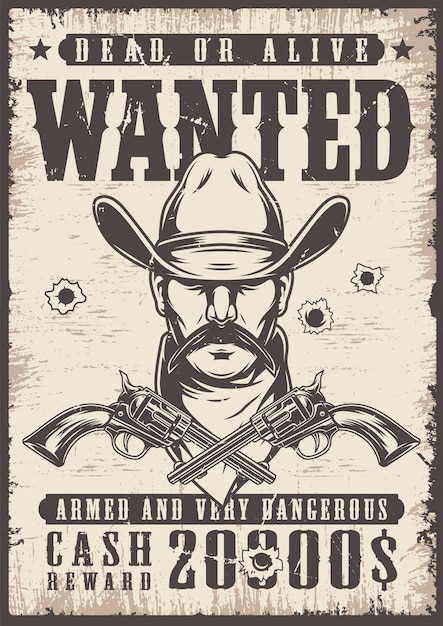This detailed wanted poster captures the essence of the old-western style with a hand-drawn, black-and-white depiction of a cowboy. The cowboy, sporting a large Stetson hat with a band that obscures his eyes, has a prominent handlebar mustache and a bandana tied around his neck. His menacing and mysterious demeanor is accentuated by the way his hat casts shadows over his face. In front of him, two six-shooter pistols are crossed, adding a touch of danger to the scene.

The weathered poster is predominantly beige with scattered off-white and light brown hues, giving it an aged appearance. A black outline frames the entire poster. At the top, bold white text within rounded rectangles declares "Dead or Alive" and "Wanted," flanked by black stars. Three distinct bullet holes pierce the poster—one on the left and two on the right—contributing to its rough, battle-worn look.

Beneath the image of the cowboy, another set of white text within a rectangle warns, "Armed and Very Dangerous," followed by bold lettering that reads "Cash Reward." The tempting amount of "$20,000" is printed beneath, with one of the zeroes punctuated by a bullet hole, reinforcing the perilous nature of the wanted individual.

Overall, this stylized, artistic piece embodies the spirit of the wild west and serves as an eye-catching decoration, perfect for adding a rugged, nostalgic touch to any setting.